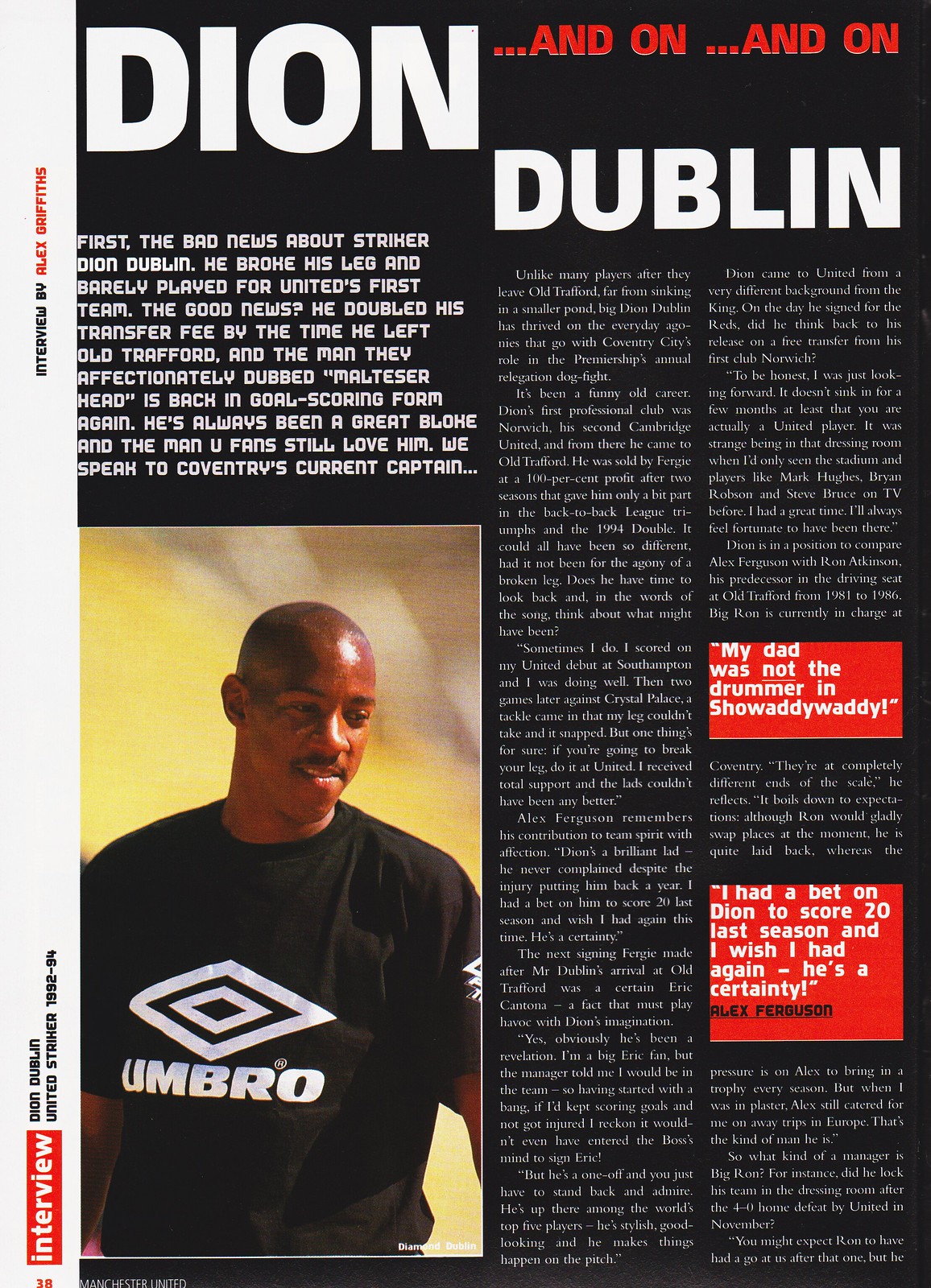The image appears to be a magazine cover featuring an interview with Dion Dublin, emphasizing his return to form in football. At the top of the page, in white text, it says "Dion," with "Dublin" on the right and "and on and on" in red on the top right. The left-hand paragraph discusses his career, mentioning how Dublin suffered a leg injury that limited his appearances for Manchester United's first team. Despite this setback, he managed to double his transfer fee by the time he left Old Trafford. The text fondly refers to him as "Malteser Head" and highlights that he's back to scoring goals, maintaining his status as a beloved figure among ManU fans.

The right-hand paragraph contrasts his successful post-United career with others who struggle in smaller leagues. Below this section, there is a photograph of Dion Dublin, a black man who appears to be in his late 20s or early 30s, wearing a black t-shirt with a white Umbro logo. A white banner nearby indicates that this is indeed an interview. Additional notable quotes in larger white text sections include "My dad was not the drummer in Showaddywaddy" and "I had a bet on Dion to score 20 last season and I wish I had again, he's a certainty," underscoring his charm and consistent performance. The background of the cover is black, which makes the text and images stand out sharply.